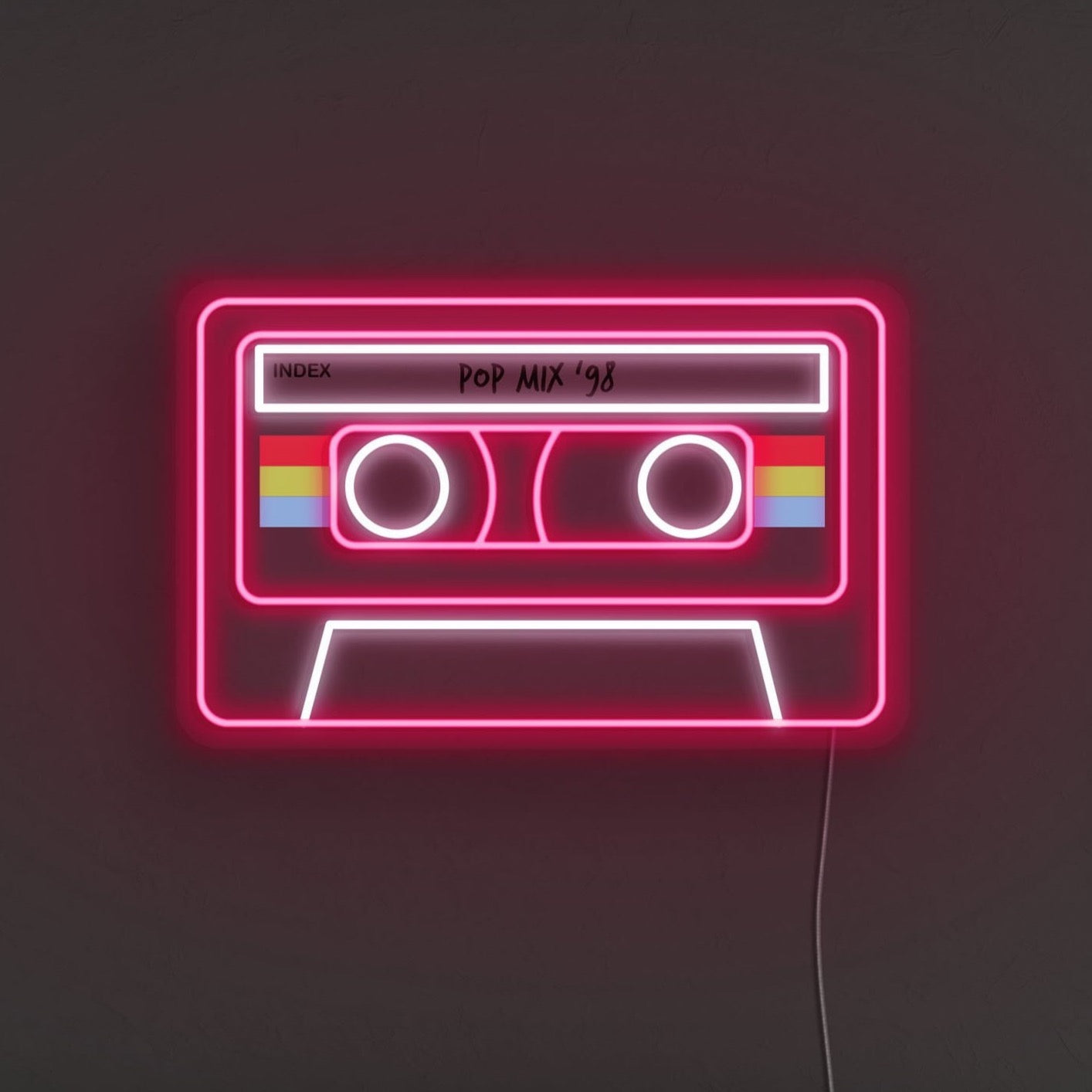The image is a striking piece of neon pop art, centered around a bright pink neon outline of a cassette tape. The cassette tape is meticulously detailed with white neon circles representing the tape reels at the center. Surrounding these reels is a pink neon rectangle, adding depth and character. On either side of this central window are three vivid horizontal stripes: red on top, lime green in the middle, and blue on the bottom, enhancing the retro vibe. The top label area, outlined in white neon, displays "Index Pop Mix 98" in a handwritten, black script. The background features a gradient of gray with pink hues emanating from the neon light, giving it a slightly ethereal glow. Adding to its realistic appeal, a wire is visible at the bottom right corner, suggesting it's a light-up sign that can be plugged into the wall. The entire composition, set against a black backdrop, exudes a modern, eye-catching aesthetic ideal for music lovers or as a stylish piece for a podcast studio.